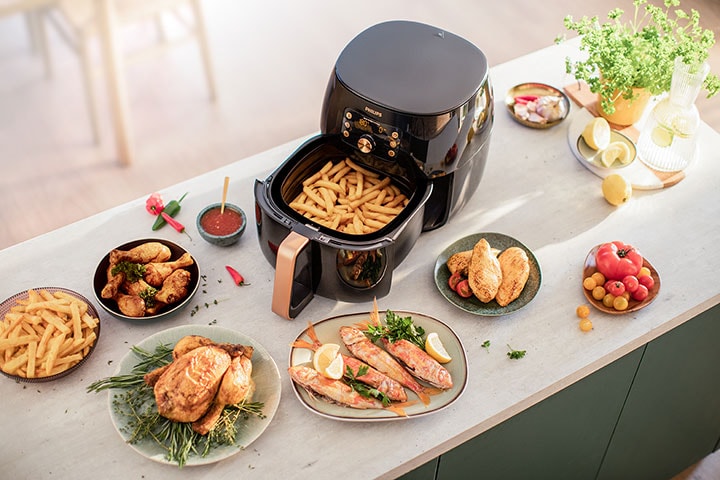This overhead image captures a vibrant, well-set kitchen island with a white countertop and contrasting forest green cabinets. Dominating the scene is a gleaming black Philips air fryer, centrally positioned and open to reveal French fries inside. Surrounding the air fryer, a culinary feast is arranged: on the left, chicken drumsticks glazed with a sauce and accompanied by a medley of red and green peppers, alongside a small bowl of red sauce. Below, a whole roasted chicken sits atop a bed of fragrant greenery, exuding a golden-brown hue indicative of perfect roasting. To the right, a plate showcases a striking reddish-orange cooked fish, garnished with fresh lemon wedges and sprigs of green parsley. Adding to the color palette is a yellow-gold plate brimming with a mix of red and yellow tomatoes. Completing the summer-like ambiance is a pitcher of water with floating lemon or lime slices, suggesting a refreshing touch, while flowers subtly enhance the daytime setting. The image, viewed from above, emphasizes the inviting and colorful array of dishes, making the air fryer the center of this delightful and diverse meal scene.